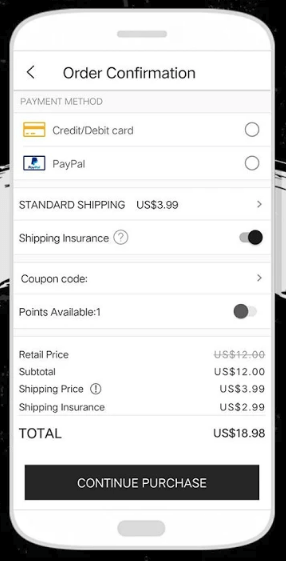The image is a screenshot showing an order confirmation page, characterized by its structured layout and clear contrasts. The top and bottom portions of the screenshot are set against a black background, while the middle section features a white background with black text. 

At the top, the text "Order Confirmation" is prominently displayed with an arrow pointing to the left, suggesting a navigation option. Below this, in gray text, "Payment Method" is stated, accompanied by an icon of a credit card to its right, followed by the text "Credit/Debit Card." Beneath this section is the PayPal logo with "PayPal" written to its right.

Further down, the text "Standard Shipping US $3.99" is present, followed by "Shipping Insurance" beside a gray circle containing a question mark. To the right of this, a toggle switch indicating the insurance option is turned on. 

Next, the text "Coupon Code" appears with an arrow pointing right, suggesting a clickable link. The section also notes "Points Available: 1," with a toggle switch in the on position.

The financial details at the bottom list "Subtotal: US $12.00," "Shipping Price: $3.99," and "Shipping Insurance: $2.99." In bold text, the total amount is displayed as "US $18.98."